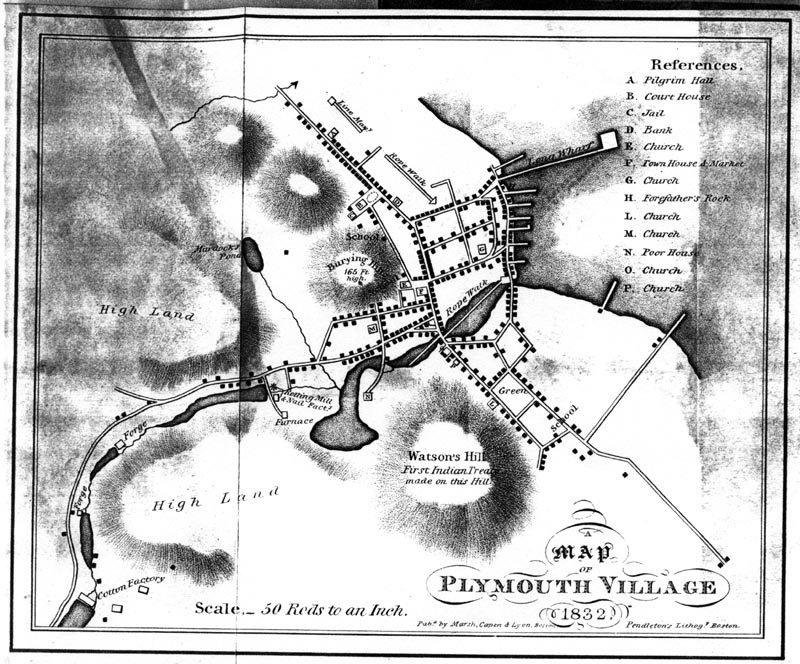This detailed black and white map appears to be a heavily photocopied image, showing Plymouth Village as it was in 1832. The quality of the image is quite poor, resembling a Xerox of a Xerox, resulting in shaded, muddy areas. 

Prominently featured in the bottom right-hand corner is the title "Plymouth Village, 1832," along with a scale reading "50 reds to an inch." The map delineates various land features, roadways, and bodies of water, marked by small squares likely representing homes or buildings. Important landmarks and areas, such as Highland on the left and below, Bering Hill in the middle, and Watsons Hill, noted as the site of the "first Indian truce," are clearly labeled.

A reference key in the top right-hand corner lists locations labeled A through P: A is Pilgrim Hall, B is Courthouse, C is Jail, D is Bank, E and G are Churches, F is Townhouse, M is Market, H is Forefathers Rock, L, M, N, O, and P are also Churches, and N is the Poor House. Notably, a significant number of these landmarks are churches, reflecting their importance in 1832 Plymouth Village. Additionally, the bottom left-hand corner of the map identifies other locations such as the Cotton Factory, Forge, and Highland.